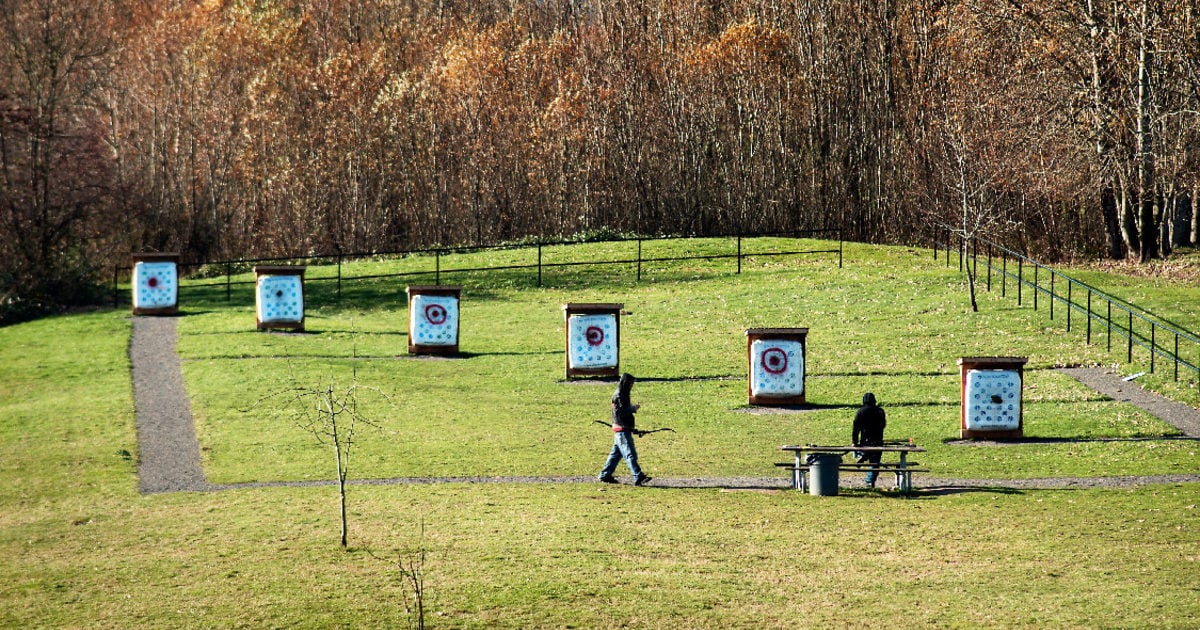This is a horizontally aligned rectangular photograph of an outdoor setting, predominantly featuring a vast grassy field that transitions into a dense, autumnal forest at the top adorned with reddish-yellow leaves. In the center of the field are two men engaged in archery. One man, dressed in jeans and a black hoodie, is walking along an L-shaped sidewalk while holding a bow. The other man is seated on a wooden picnic table, his back to the camera, with a trash can visible behind him. 

Scattered in a diagonal line across the grassy area are six targets, each with white faces adorned with red bullseyes and numerous small blue dots, set progressively further into the field. The area is bordered by a black piped fence that runs parallel to the sidewalk. This detailed scene suggests a serene, fall-time target practice session amidst nature's vibrant colors.